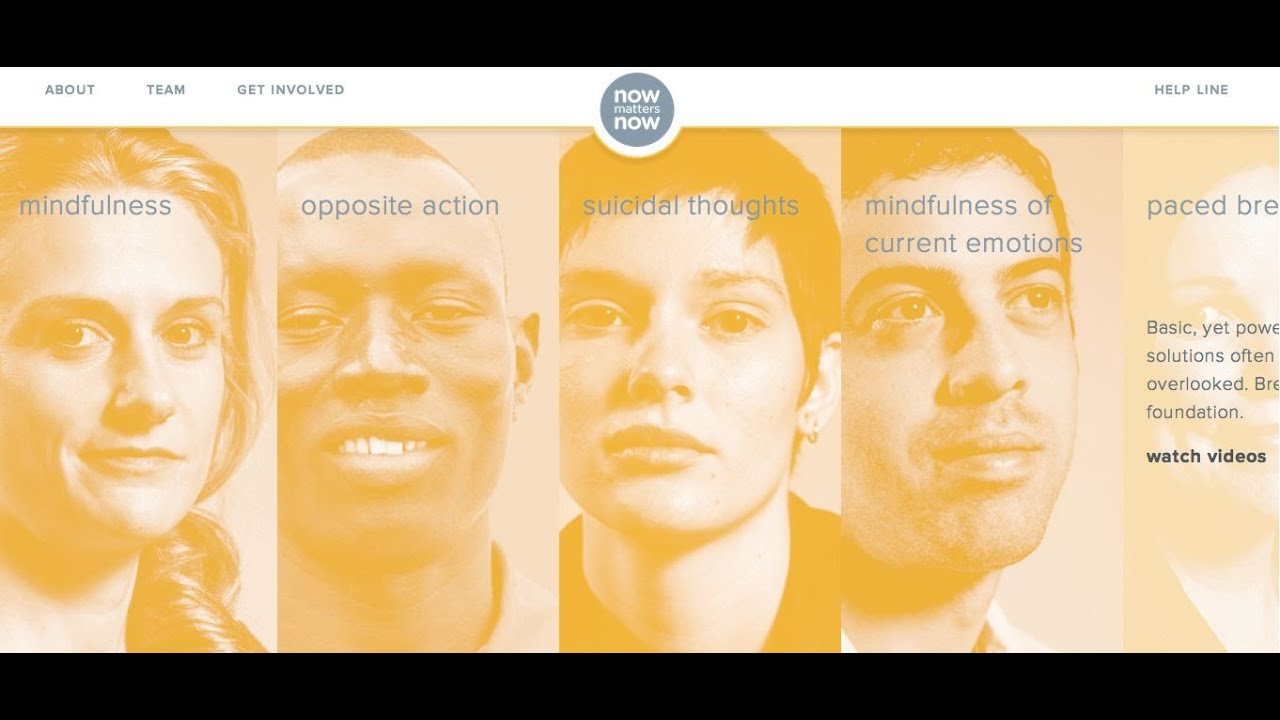This image showcases a website layout with the primary focus on the phrase "Now Matters Now," prominently displayed in a circular area at the top center. The word "Now" is presented in bright white text, while "Matters" appears in a slightly grayish-white hue, both set against a gray background within the circle. At the very top of the image, a black horizontal rectangular bar spans the width, mirrored by another bar at the bottom.

Beneath the top black bar, on the far left, three menu options are visible: "About," "Team," and "Get Involved," all rendered in grayish text. On the right side of this area, there is an option labeled "Help Line."

Dominating the central portion of the image, four distinct sections are displayed, each dedicated to specific actions. The first section, titled "Mindfulness," features an image of a woman as its background. The second, labeled "Opposite Action," includes the image of a Black man. The third section, "Suicidal Thoughts," shows a woman with black hair. The fourth and final section, "Mindfulness of Current Emotions," depicts a white man. Each of these images is overlaid with a subtle orange tint, adding a cohesive visual theme to the photo.